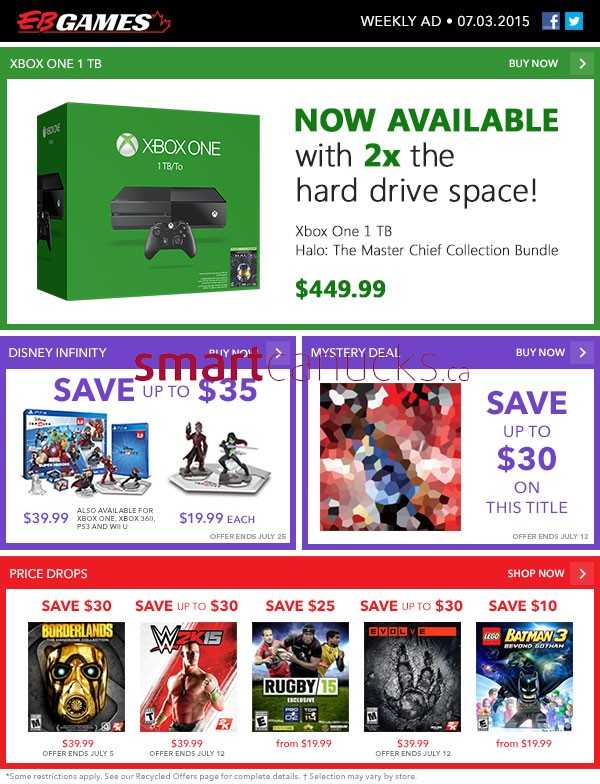**Image Caption: Detailed Overview of a Weekly Ad on EB Games**

The image is a screenshot of a weekly ad page from the EB Games website, featuring various deals on video games and consoles. The website's logo, a distinctive red and white design, is displayed prominently on the left side of the top navigation bar. On the right side of the bar, text indicates this is a weekly ad dated July 3, 2015, accompanied by social media icons for Facebook and Twitter.

Below the navigation bar, the ad content is organized into different colored boxes, each highlighting specific deals. The topmost and largest box is green, advertising the availability of the Xbox One with double the usual hard drive space, priced at $449.99.

Moving down to the middle section, there are two purple boxes side by side. The left box promotes Disney Infinity, offering savings of up to 35% on select action figures and video games, with prices listed at $39.99 and $19.99 each. The right box features a blurry, pixelated image and teases a mystery deal that promises savings of $30 on an undisclosed game or title.

At the bottom of the ad, a red rectangular box lists price drops for various video games. The featured deals include:
- Borderlands: Save $30
- WWE: Save up to $30
- Rugby 15: Save up to $25
- Evolve: Save up to $30
- Batman 3 Beyond Gotham: Save $10

To the right of these promotional boxes, a prominent "Buy Now" or "Shop Now" button is displayed, inviting users to take advantage of these offers immediately.